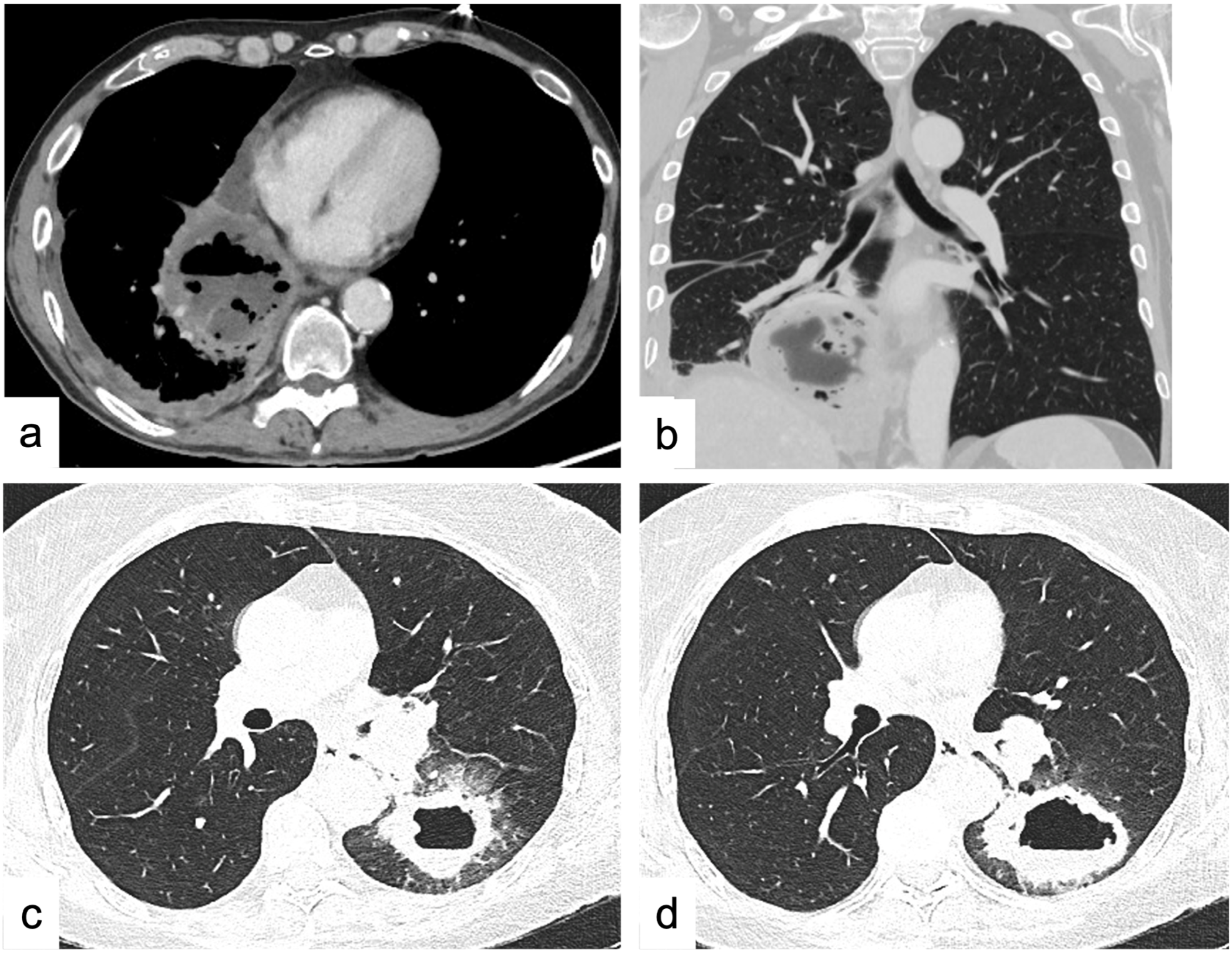This image presents a grid of four black and white medical scans, labeled A, B, C, and D, arranged in a two-by-two format with a distinct white line separating each section. Each smaller image shows a different view of body parts, likely obtained through MRI or CT scan technology. 

In the top-left quadrant (Image A), the scan reveals an oval-shaped area with dense, splattered liquid-like structures in the center, possibly an overhead view of internal organs. The top-right quadrant (Image B) displays a front view of a pair of lungs, clearly depicting the rib cage as oblong rings encircling darker lung tissue. 

The bottom-left (Image C) and bottom-right (Image D) quadrants appear to show similar images to the top-left, with dense white areas resembling the spinal column surrounded by a black backdrop and lighter gray veins or tissues. These images reflect variations in imaging techniques, emphasizing different anatomical details throughout the body.